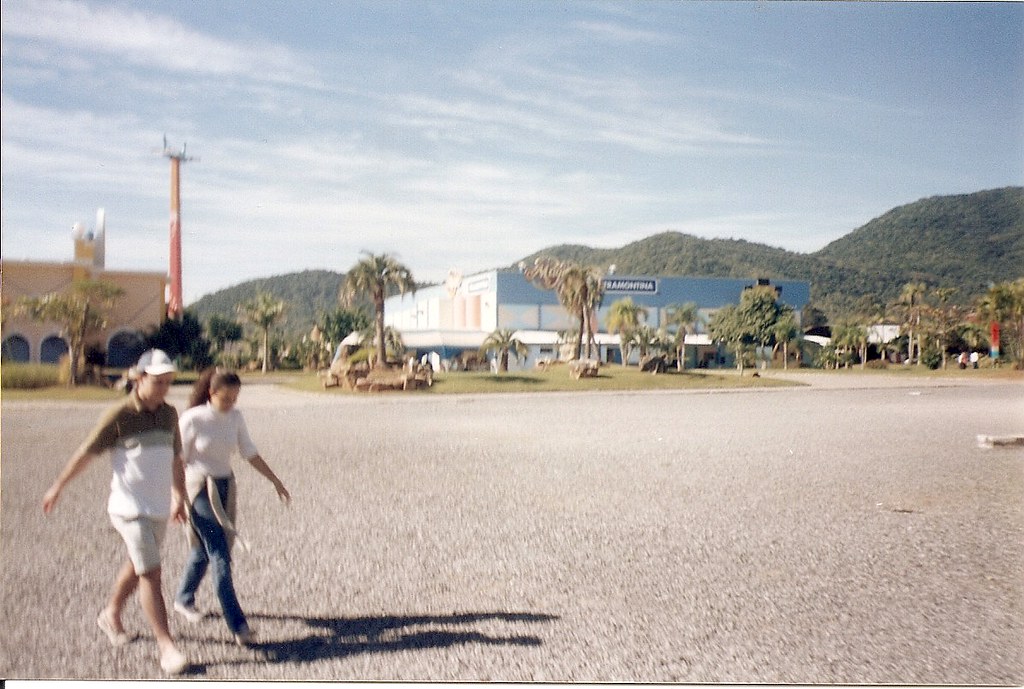In this outdoor photograph, the foreground features a gravel roadway taking up the bottom half of the image. In the bottom left corner, two individuals are walking from left to right. The person on the left is a man wearing a t-shirt with a green top section and whitish-black mixed stripes around the chest, paired with white shorts and white shoes. He also has a white hat with a black back half. The woman walking next to him on the right is dressed in a white t-shirt, blue jeans, and a white jacket tied around her waist. Her dark hair is pulled back into a ponytail. Both are looking down at the ground.

Behind them, in the middle ground, there are two distinct buildings. On the left stands a beige-colored building with arched windows, adjacent to a tall, rectangular red tower that rises into the sky. To its right is a large, squarish blue building that has a dark blue sign with white, unreadable lettering. Interspersed among the buildings and surrounding them are various trees, including some palm trees of differing heights. 

In the background, a mountain range covered with brush and dense trees stretches across the horizon. Above the mountains, the sky is blue with scattered white clouds, completing the picturesque setting. The clarity of the photo is somewhat reduced, giving it a grainy texture. Shadows cast on the ground suggest the time of day, adding depth to the scene.